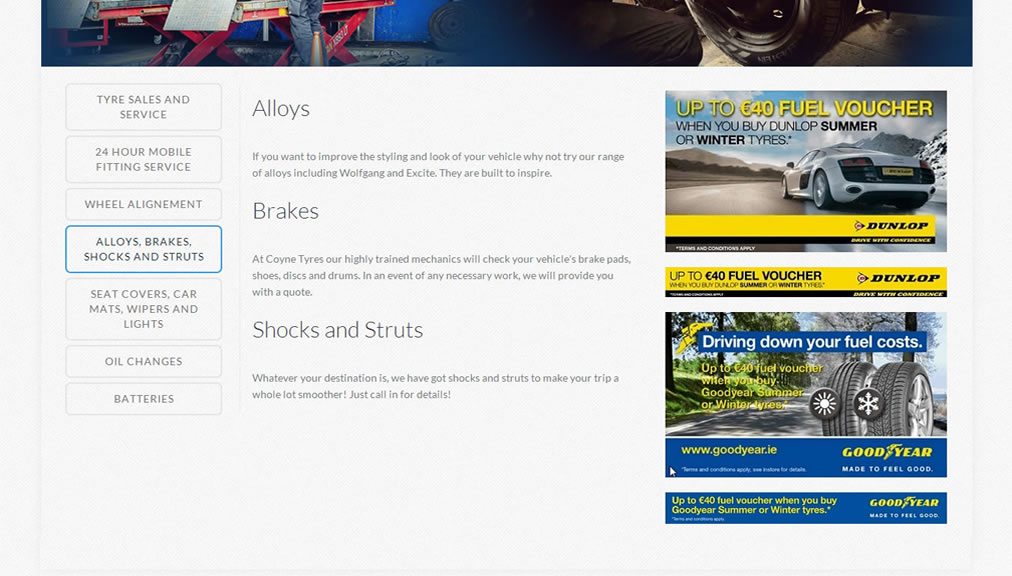This image showcases a portion of a desktop website, presumably for Coyne Tyres. The web address, browser, and operating system are not visible. The picture includes a fragment of a workshop scene and a partially visible car tire. 

On the left side of the image, there are several service options presented in a blackish-gray font within rectangular boxes, all in uppercase letters. The options include:
- Tyre Sales and Service (tire spelled as T-Y-R-E)
- 24-Hour Mobile Fitting Services
- Wheel Alignment
- Alloys, Brakes, Shocks, and Struts (highlighted in blue)
- Seat Covers, Mats, Wipers, and Lights 
- Oil Changes
- Batteries 

In the central area, the focus shifts to details about various services:
- "Alloys: If you want to improve the styling and look of your vehicle, why not try our range of alloys including Wolfgang and Excite. They are built to inspire."
- "Brakes at Coyne Tyres: Our highly trained mechanics will check your vehicle's brake pads, shoes, discs, and drums. In the event of any necessary work, we will provide you with a quote."
- "Shocks and Struts: Whatever your destination is, we have got shocks and struts to make your trip a whole lot smoother. Just call for details."

On the right side of the page, two advertisements are visible:
1. An ad featuring a silver hot rod promoting a €40 fuel voucher when purchasing Dunlop summer or winter tyres.
2. Another similar promotion for Goodyear with the tagline "Made to Feel Good" and details about the €40 fuel voucher when buying Goodyear summer or winter tyres. The URL www.goodyear.ie is also mentioned.

Assuming this is Coyne Tyres' website, it highlights their comprehensive automotive services and various promotional offers for tyres.